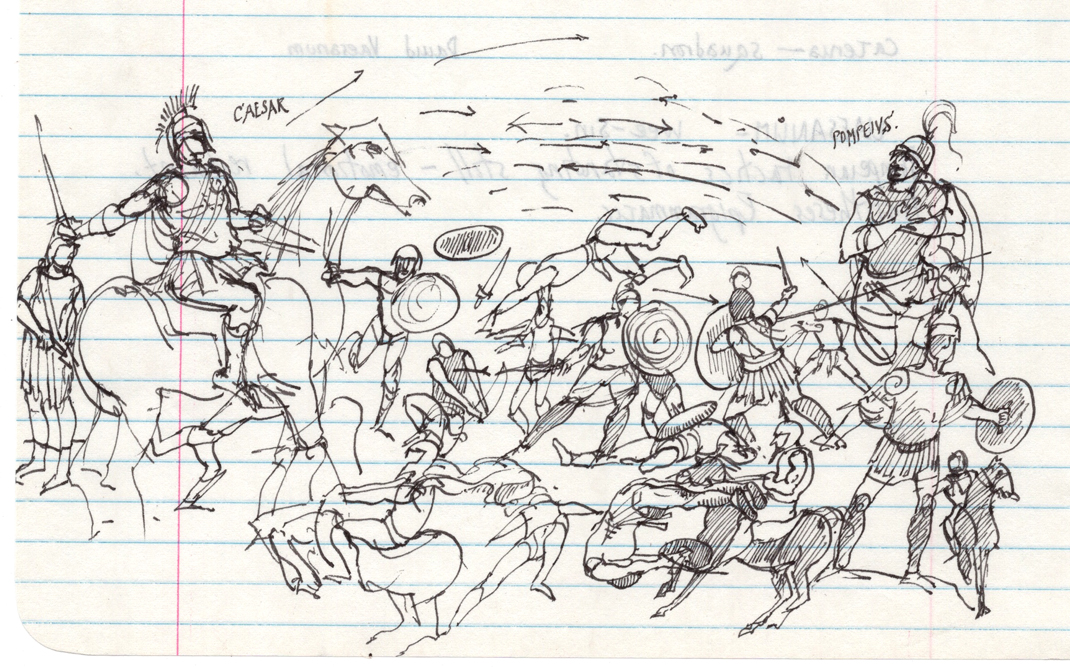This detailed drawing is crafted on an older piece of college-ruled notebook paper, characterized by its off-white background and thin blue horizontal stripes. The rectangular image, approximately six inches wide and three inches tall, features a red vertical stripe about an inch from the right edge. The artist used black ink to illustrate an intense Roman battle scene. On the left side, a large figure labeled "Caesar" is depicted riding a horse, adorned in traditional Roman armor. On the opposing right side, another figure labeled "Pompeius" stands or possibly rides a horse as well, mirroring Caesar. The sky is filled with flying arrows, while approximately 20 soldiers engage in combat on the ground, wielding shields and swords. The meticulous detailing of the soldiers and the dynamic array of arrows convey the chaos of battle, with Caesar positioned slightly higher, perhaps implying his commanding presence over Pompeius.